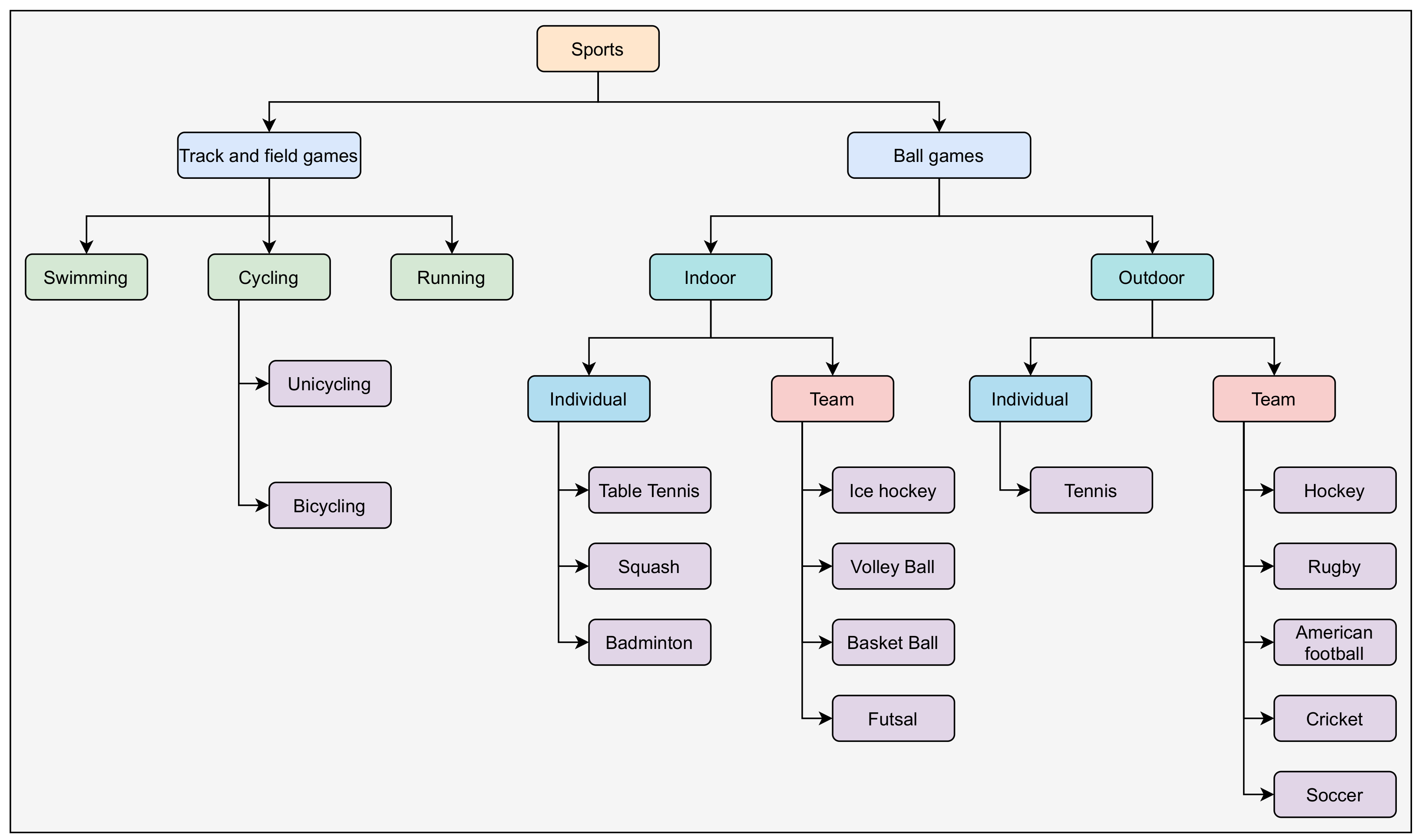The image is a detailed flowchart of sports against a simple grayish, pale purple background. At the top of the chart, "Sports" is prominently displayed in orange. From there, it branches into two blue sections: "Track and Field Games" on the left and "Ball Games" on the right.

Under "Track and Field Games," further subdivisions include "Swimming," "Cycling," and "Running." The "Cycling" category itself branches into two activities: "Unicycling" and "Bicycling."

The "Ball Games" section branches into "Indoor" and "Outdoor" categories. Each of these is further divided into "Individual" and "Team" games. In the "Indoor" individual section, listed games include "Table Tennis," "Squash," "Badminton," with team sports such as "Ice Hockey," "Volleyball," "Basketball," and "Foosball." The "Outdoor" individual section includes "Tennis," whereas team sports comprise "Hockey," "Rugby," "American Football," "Cricket," and "Soccer."

The chart provides a comprehensive breakdown of various sports categories, clearly delineated by color-coded sections, making it an effective visual representation of sports activities available, perhaps at an educational institution.